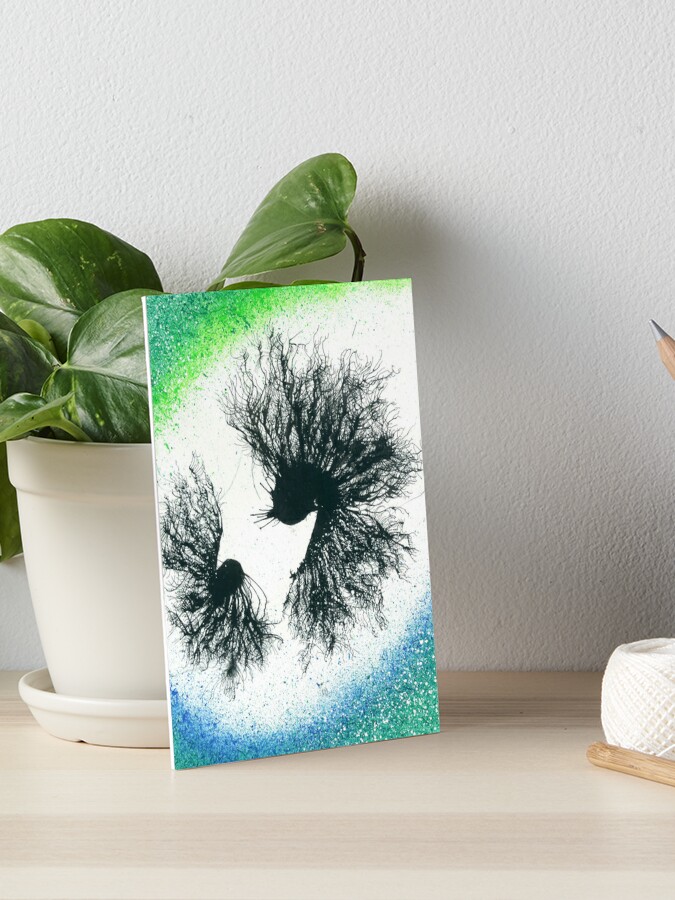The photograph captures a serene, minimalist display set against a slightly textured, off-white wall with a hint of tan trim. The scene centers around an off-white ceramic pot housing a lush, deep green devil's ivy, also known as pothos, with its glossy leaves cascading gently. Leaning against the pot is an abstract painting, the focal point of the arrangement.

The painting is characterized by its unique composition: the middle of the canvas is predominantly white, adorned with two black, abstract shapes reminiscent of delicate, wispy angelfish or bettafish, or alternatively, dandelion seeds dipped in black paint and rolled across the surface. Surrounding these central forms, the painting transitions into a medley of speckled blue and green hues. The upper left corner is more vibrant with greens while the bottom right corner displays shades of blue, blending to create an intriguing visual texture.

To the right of the painting sits a spool of white twine, adding an element of rustic simplicity to the composition. On the light, pale whitish-brown wooden surface, the tip of a pencil peeks into view halfway up the right edge, lending a subtle touch of practicality to the otherwise artistic and organic display.